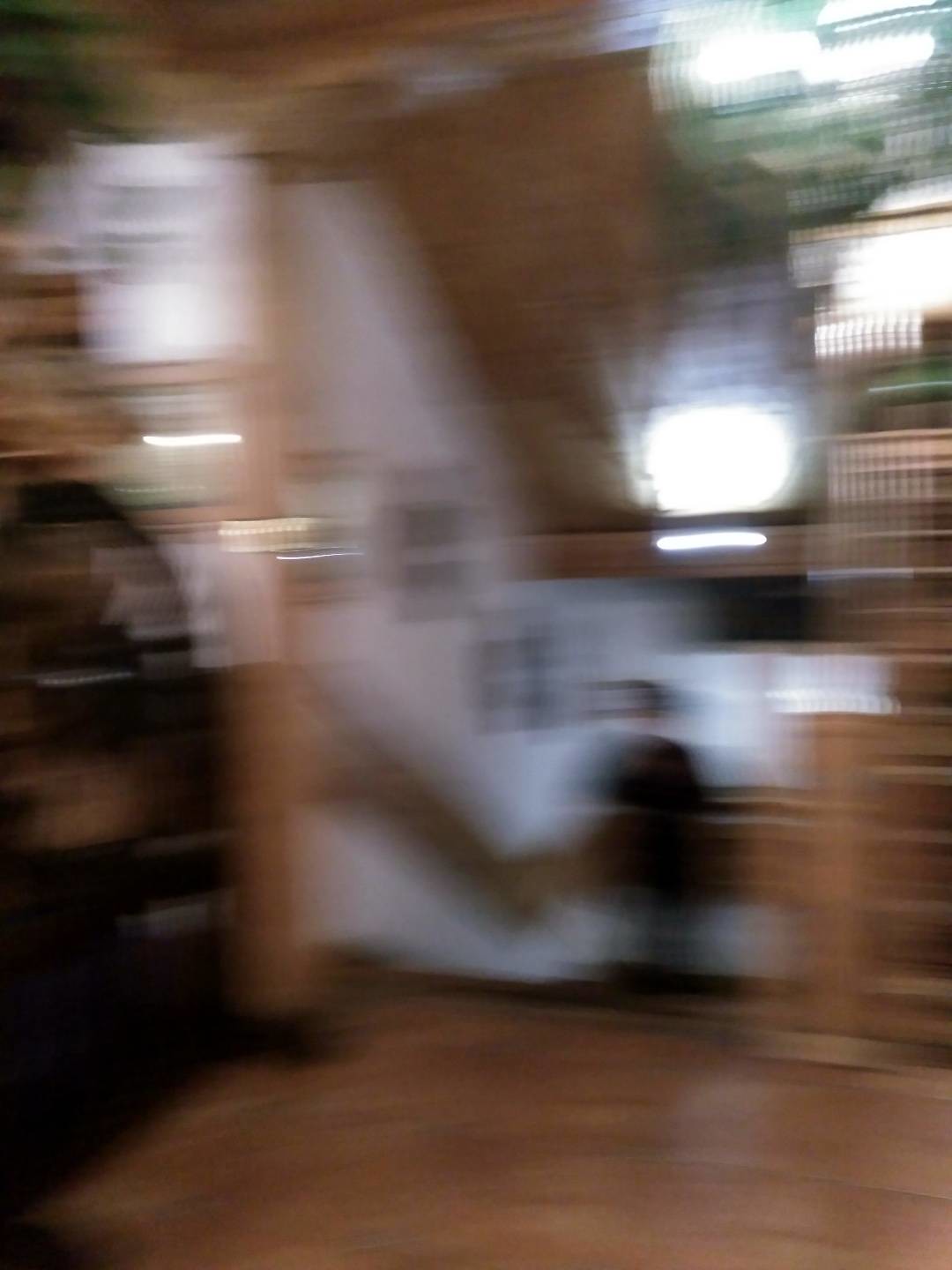A blurry image of what appears to be a kitchen corner. Despite the lack of clarity, you can discern a section of the room that likely contains kitchen elements. In the upper left-hand side, a window is faintly visible. Another window is noticeable towards the upper center-right side. On the far right, there appears to be shelving, and the floor is seemingly covered in linoleum. The overall scene suggests an indoor setting, probably a kitchen, even though the blurriness makes it difficult to identify specific objects.